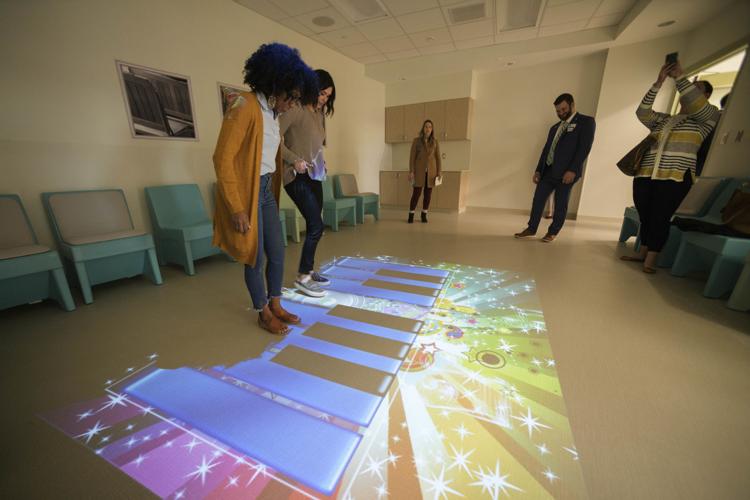In a beige-colored room, five people are standing around in a spacious circle. Two women are at the center, positioned on top of a vibrant, virtually projected piano keyboard on the floor. The keys, which come in shades of purple, blue, and black, are surrounded by a whimsical sunburst pattern featuring yellow, gold, red, and other colors. These women appear poised to play music with their feet on the simulated instrument. To the side, a man in a striped sweater stands with his phone held high, seemingly recording the action. Looking on is a man in a suit jacket with a name tag, focused on the projected piano. Another woman, dressed in a knee-length coat, stands further back, holding a white object. Blue chairs line the back wall, offering seating for those waiting or observing. The scene is both lively and curious, with the mix of technology and interactive play grabbing everyone's attention.